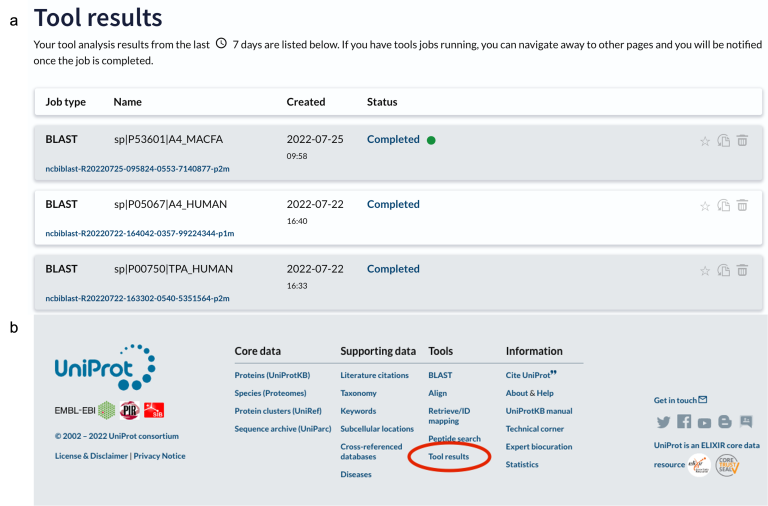This is a detailed screenshot of a website displaying tool results. In the top left corner, black text reads "Tool Results," and immediately below that, another line states, "Your tool analysis record or results from the last seven days are listed below. If you have tool jobs running, you can navigate away to other pages, and you'll be notified once the job is completed."

The table is organized into four columns with headers: "Job Type," "Name," "Created," and "Status." Each row beneath these headers represents a job entry.

- **Job Type:** All entries list "BLAST," written in capitalized black text.
- **Name:** The first entry reads "SPIP53601A4 MACFA," and the second entry is "SPIP53601A4 HUMAN."
- **Created:** The first job was created on July 25, 2022, and the second on July 22, 2022.
- **Status:** [Status would be detailed, but is missing in the provided text]

The rows visibly distinguish between the job names and creation dates, presenting a clear record of each tool's activity within the specified timeframe.